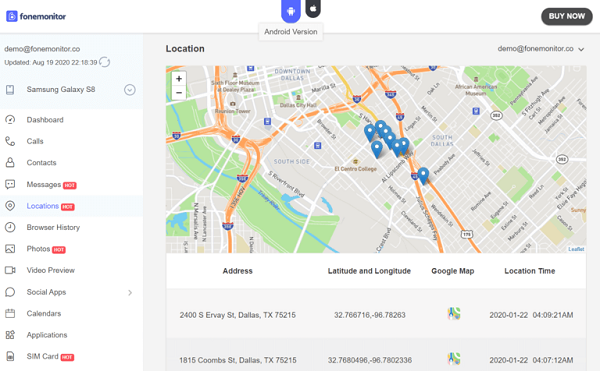**Detailed Caption:**

The image is a screenshot of a digital interface from a monitoring application, likely accessed through a website or an app, displayed in landscape orientation. The interface features a clean, white header at the top. On the top left of the header, the application's name, "fone monitor" (all lowercase and in black text), is accompanied by a small blue square logo. In the center of the header, there are two selectable tabs: one for the "Android version," marked by a blue U-shaped icon with a white Android robot, and another for the "iPhone version," represented by a black icon with a white Apple logo. The Android version is currently selected. On the top right, there's a prominent black, oblong button labeled "Buy Now."

Beneath the header, on the left side of the screen, there's a vertical column featuring user information and device options. At the top of this column, there's an email address, "demo@phonemonitor.co," along with a last updated timestamp of "August 19th, 2020." Below this, a list of 13 menu items is displayed, starting with the device name "Samsung Galaxy S8." This item includes a dropdown arrow indicating it can be expanded, which reveals further options such as:

1. Dashboard
2. Calls (with a phone handset icon)
3. Contacts
4. Messages (marked with a "NEW" red flag)
5. Locations (marked with a "NEW" red flag and highlighted in pale blue, indicating it’s currently selected)
6. Browser History
7. Photos (marked with a "NEW" red flag)
8. Video Preview
9. Social Apps (with a speech bubble icon)
10. Calendars
11. Applications
12. SIM Card (marked with a "NEW" red flag)

The main section to the right displays a map centered on the selected "Locations" option. This street map features blue location points and beneath it, detailed information about specific locations are provided. Each entry includes the address (e.g., "2400 South Ervay Street, Dallas, Texas, 75215"), latitude and longitude coordinates, a small Google Maps thumbnail, and location time stamped "2020-01-22 04:09:21 AM."